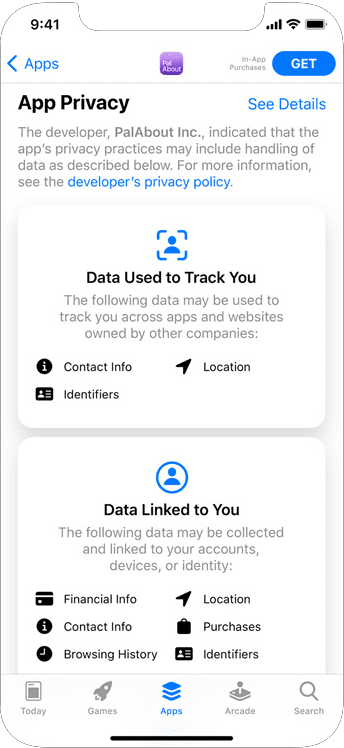This smartphone screenshot features a predominantly white background, typical of an app's information page. In the upper right corner, standard status icons are visible, indicating a fully charged battery, active Wi-Fi, and wireless connection signals. The upper left corner displays the time in black font as "9:41", without specifying a.m. or p.m.

Directly below the time, in blue font, is the label "Apps" accompanied by a left-pointing arrow, hinting at navigation options. Centrally positioned on the screen is a small purple rectangle, seemingly a logo, containing the barely legible words "pay" and "about". To the right of this logo is a blue rectangle with rounded corners, bearing the word "Get" in white, suggesting a clickable button to install the app.

The headline "App Privacy" dominates the middle of the screen in large font. Beneath it, in gray text, the message reads: "The developer, Pal About Inc., indicated that the app's privacy practices may include handling of data as described below. For more information, see", followed by a blue hyperlinked text "Developer's Privacy Policy".

The next section, labeled "Data Used to Track You" in a prominent font, details that the app may track: Contact Info, Identifiers, and Location. Following this, another section titled "Data Linked to You" lists categories of personal data that are connected to the user, which include: Financial Information, Contact Info, Browsing History, Location, Purchases, and Identifiers.

At the bottom of the screen, a footer displays iconographic navigation options for different sections: Today, Games, Apps, Arcade, and Search, arranged from left to right.